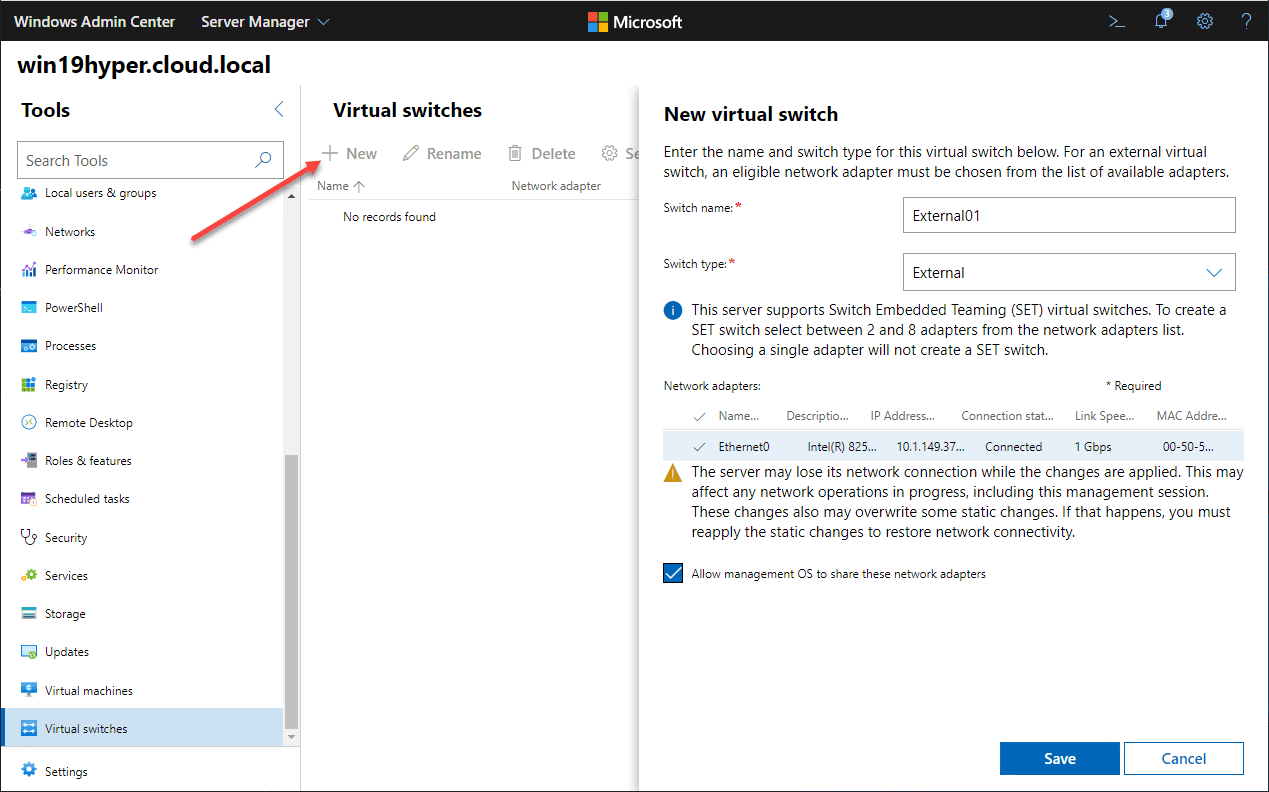This web page showcases the Microsoft Windows Admin Center Server Manager interface. At the top, there is a thin black bar featuring the Microsoft logo. Currently, the web menu is exploring the server "win19hyper.cloud.local." On the left side of the page, the toolbar is present, with the "Virtual Switches" option highlighted. This selection has revealed a detailed configuration panel in the center of the screen, allowing the user to create and manage virtual switches. The configuration panel provides fields for entering the switch name, selecting the switch type, and specifying the network Ethernet location. Users can make their entries and save the changes via the options provided in this sub-window.